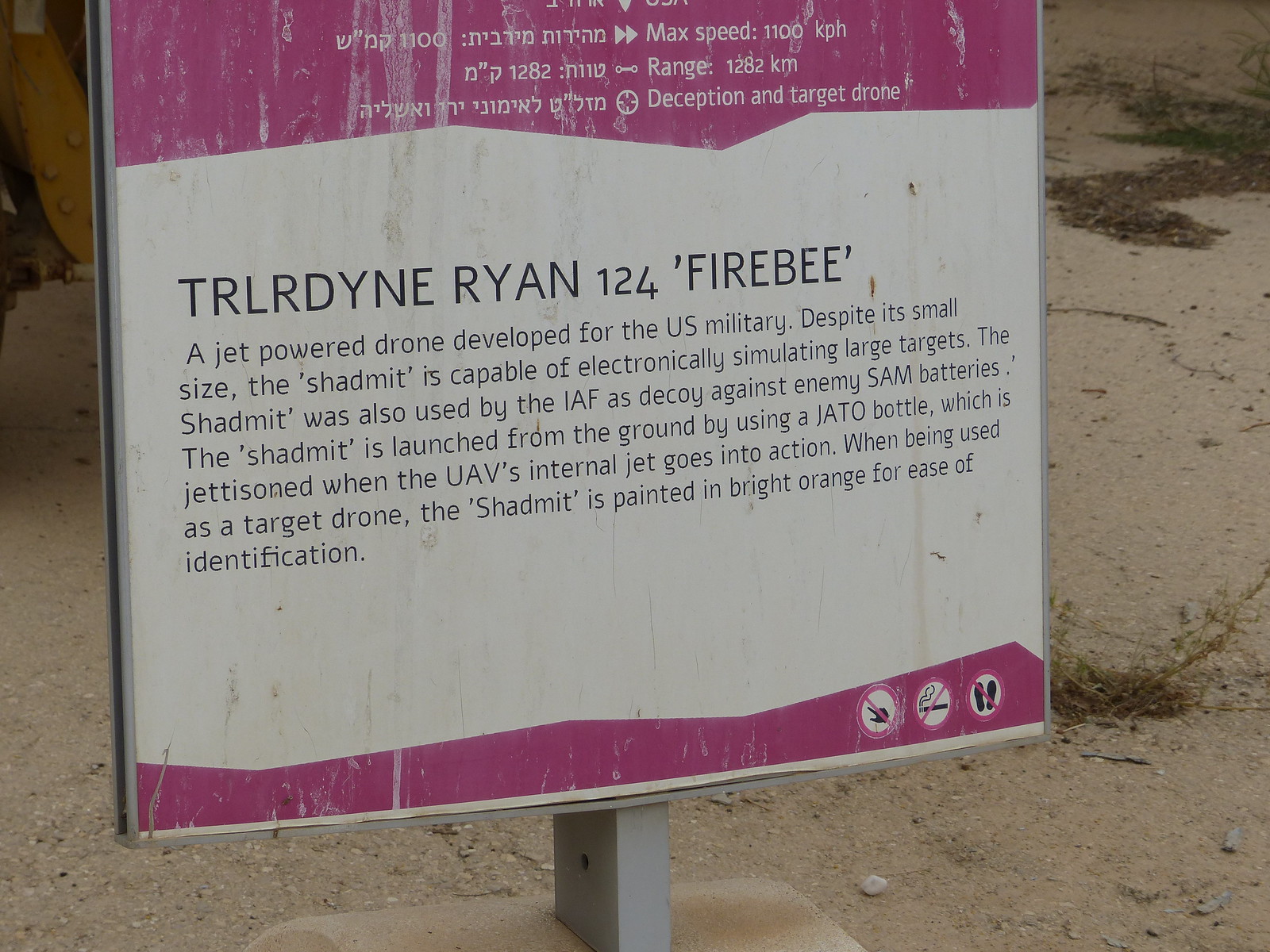The image depicts a worn sign, prominently centered and mounted on a small concrete platform amidst a sandy, desert-like terrain with scattered patches of vegetation and rocks. The sign features text in both English and Hebrew, with a title reading "Turlodyne Ryan Firebee." The description below details a jet-powered drone developed for the U.S. military, known as the Shadmint. Despite its small size, the Shadmint can electronically simulate large targets and has been used by the IAF as a decoy against enemy SAM batteries. The Shadmint is launched from the ground using a JATO bottle, which is jettisoned when the UAV's internal jet activates. When serving as a target drone, it is painted bright orange for ease of identification. The sign is surrounded by symbols indicating no smoking and no trespassing. The image is taken outdoors in what appears to be the middle of the day, emphasizing the pink, white, and tan hues of the sign against the dry, earthy backdrop.